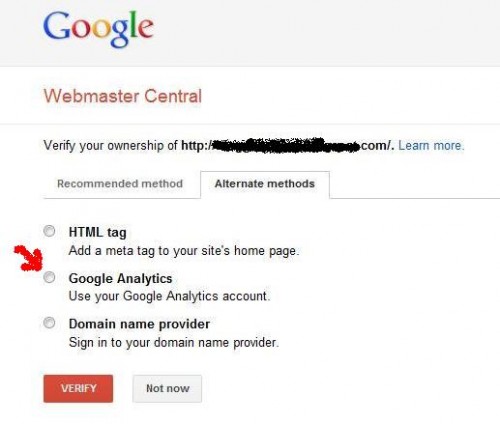This is a vertically-oriented image, resembling a smartphone or computer screen interface, depicting a Google verification page. The background is predominantly white, with a medium gray rectangular box at the top displaying the Google logo in its iconic multicolored format. Below this, the background transitions to white with the heading "Webmaster Central" in orange, delineated by a separator line.

Underneath, in black text, it reads "Verify your ownership of," followed by a web address obscured by black scribbles. A blue "Learn more" button is positioned nearby. The interface highlights two sections: "Recommended method" and "Alternate methods," with the latter being the selected option, indicated by bold text. The three alternatives within this section include:

1. **HTML tag**: Add a meta tag to your site's homepage.
2. **Google Analytics**: Use your Google Analytics account.
3. **Domain name provider**: Sign in to your domain name provider.

Each method is accompanied by an unselected circular radio button. A prominent red arrow points to the circular button next to "Google Analytics." At the bottom, an orange "Verify" button and a gray "Not now" button offer action choices.